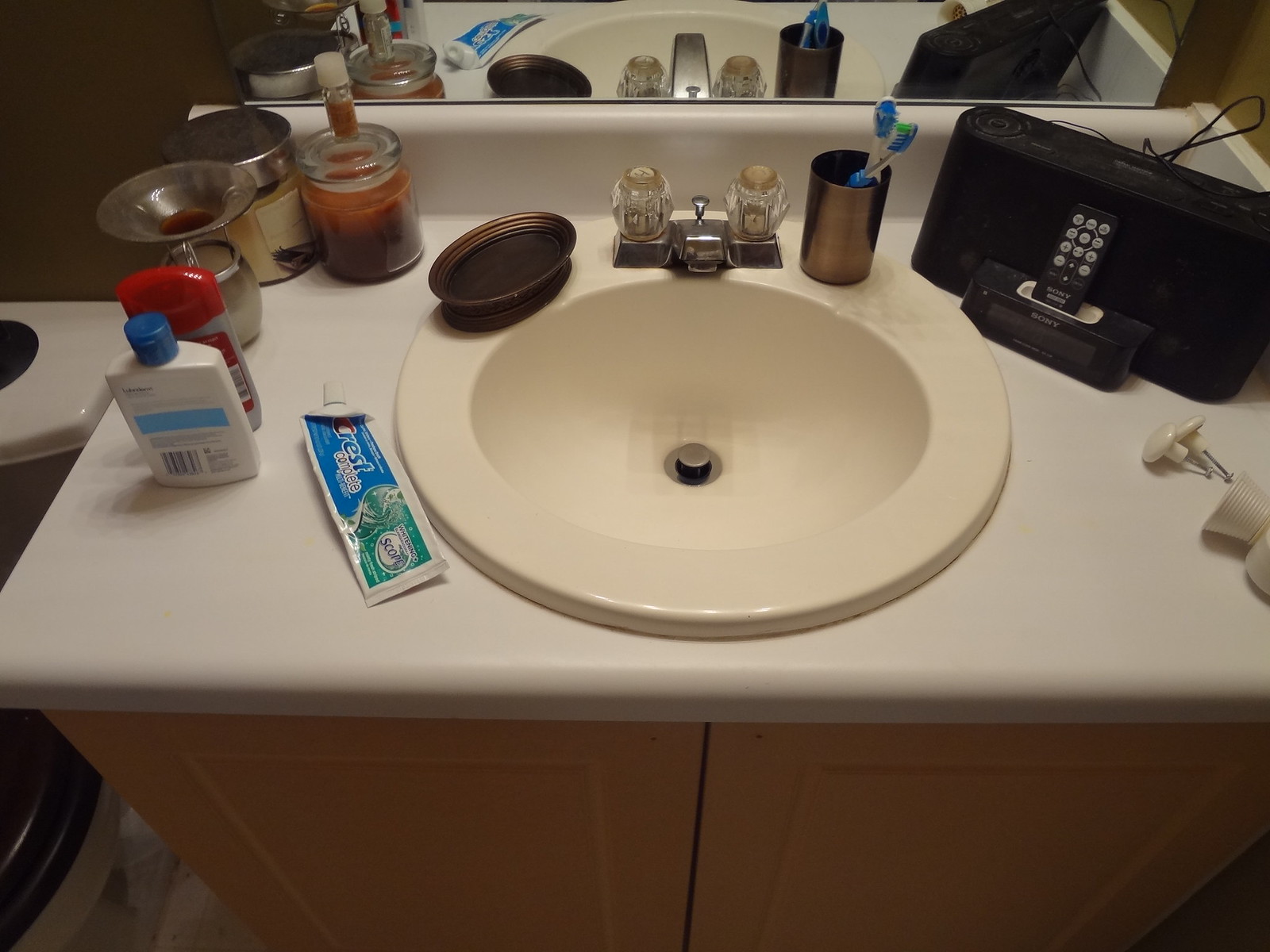This image depicts a bathroom vanity with a beige basin featuring two clear plastic handles on an antique silver-tarnished faucet. Accentuating the basin are a bronze or antique brass soap holder and toothbrush holder. The countertop is cluttered with a nearly empty blue and white tube of Crest toothpaste, a deodorant stick, various tubes possibly containing soap or lotion, and a couple of scented candles. A black speaker system or radio with a remote resting on top is also visible, along with its cords plugged into an unseen outlet. Above the basin is a mirror, while below the vanity are light wood-colored cabinets.